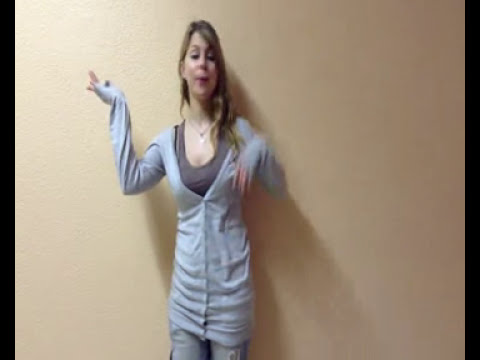The image portrays a young woman in her early twenties, poised against a wall and seemingly engaged in an artistic performance. She is dressed in a layered outfit comprising a light gray knee-length sweater over a dark gray blouse, paired with dark jeans. The woman's light brown hair cascades over her left shoulder. Her arms are expressive; the right arm extends away from her body with the palm facing up, while the left arm is held out in front with the palm pointing down, indicating dynamic movement. Her lips appear pursed as though she is singing. The overall impression is that she is dancing, possibly for a social media platform like Instagram, TikTok, or Reddit, blending fluid arm motions with a potential vocal performance.